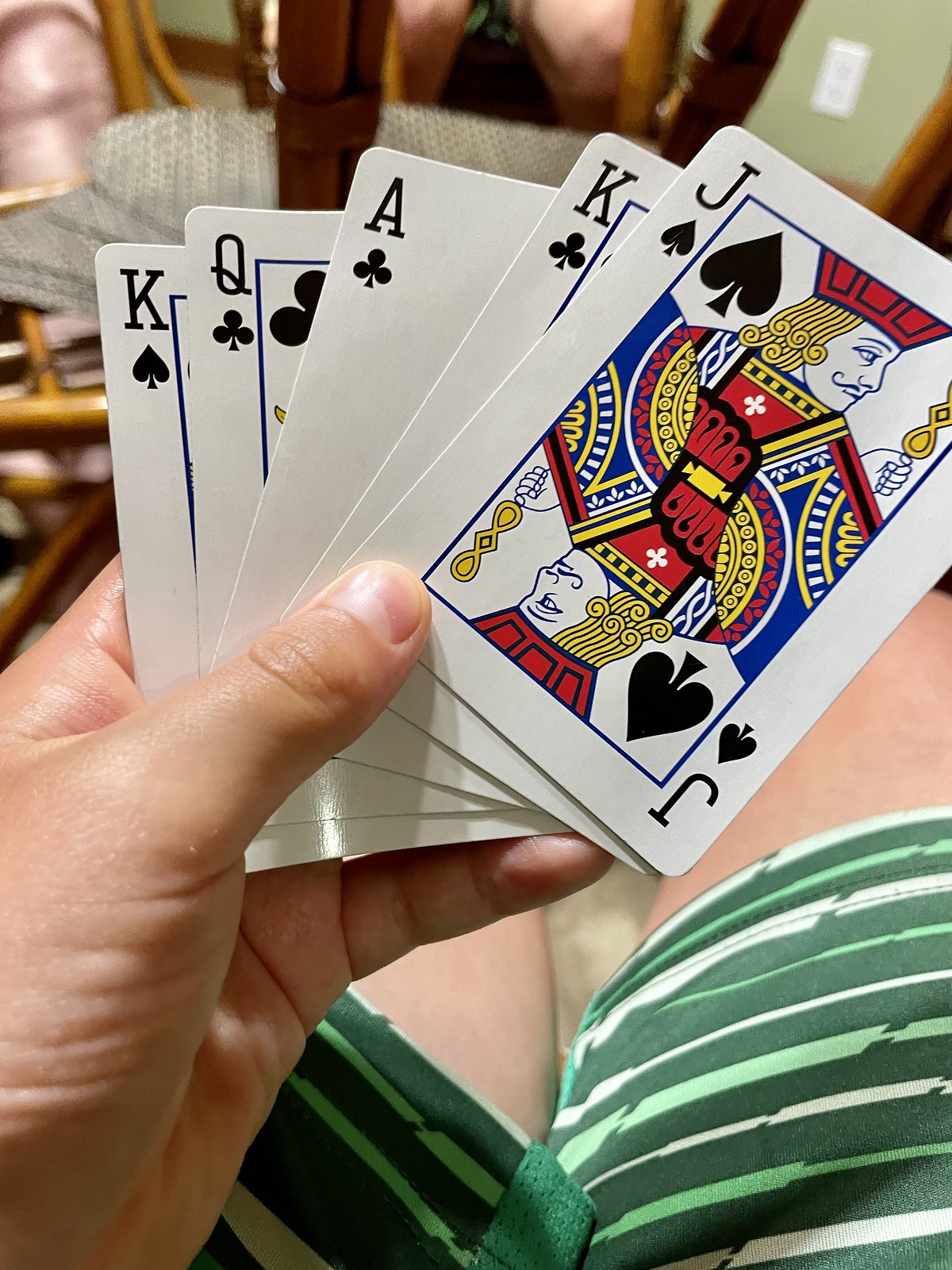In the photograph, a left hand, identifiable by its light-skinned, somewhat masculine appearance, holds a fanned-out hand of playing cards. The cards arrayed from left to right are the King of Spades, the Queen of Clubs, the Ace of Clubs (slightly more revealed than the others), the King of Clubs, and the Jack of Spades. The playing cards feature a white background with black text, except for the Jack, which displays a colorful illustration. 

The backdrop of the image is slightly blurred. In the background, there is a wooden chair with gray woven padding on the seat. The area beyond includes elements of wood, patches of pink, and a white wall accompanied by light brown woodwork. Beneath the playing cards, a fabric with green and ivory stripes can be seen, possibly shorts that someone is wearing. Additionally, a knee of white skin peeks out from beneath the striped fabric. The composition blends elements of everyday life with the moment of holding a hand of cards, adding to the image's overall narrative.